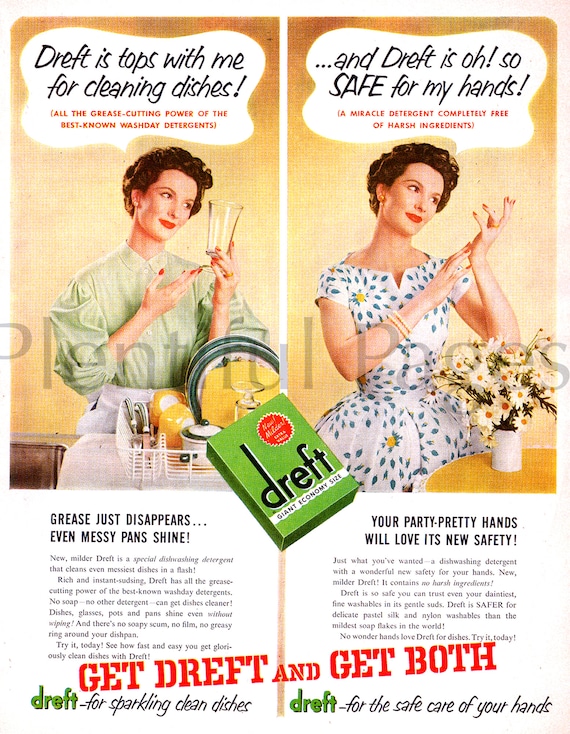This vintage marketing flyer for DREFT, likely from the 1940s or 1950s, showcases the effectiveness and gentleness of the cleaning detergent through a compelling visual narrative. The horizontal image, about the size of a piece of paper in portrait view, features a housewife depicted twice—once on the left and once on the right—emphasizing the dual benefits of the product.

On the left side, the woman, styled with short dark hair and bright red lipstick, dons a white dress with blue polka dots. She stands in a kitchen setting, proudly holding up a spotless, shiny glass cup in her left hand, while her right hand points to it. The surrounding dish tray, filled with drying dishes, underscores the product's grease-cutting power. A dialogue box above her states, "DREFT is tops with me for cleaning dishes. All the grease-cutting power of the best known wash day detergents."

On the right side, the same woman appears in the same pose, but this time is positioned at a dining table adorned with a bouquet of flowers. Her left hand is empty and gently clasped by her right hand, indicating she no longer needs to stress over washing dishes. Above her head, another dialogue box reads, "And DREFT is oh so safe for my hands, a miracle detergent completely free of harsh ingredients." The radiant and content expression on her face in both images highlights the product's ability to deliver sparkling clean dishes while being gentle on her hands.

Centrally, a box announces "DREFT, giant economy size," reinforcing the product's value, while the bottom third of the flyer contains additional marketing content in bold red lettering that urges readers to "Get DREFT and get both." This comprehensive depiction assures the consumer of DREFT's effectiveness in cleaning and safety for personal care.